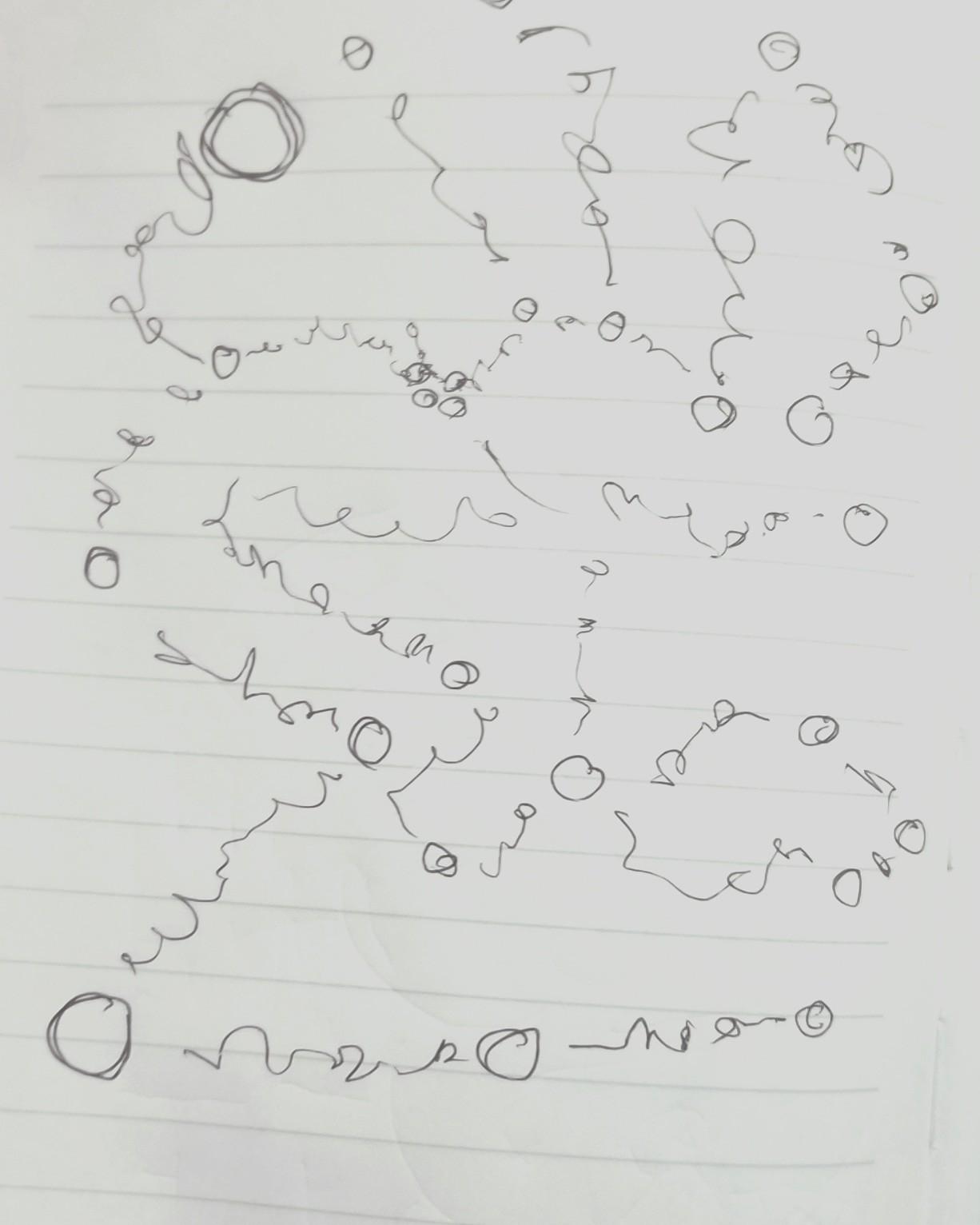This photograph captures a piece of white, lined paper with light gray horizontal lines. The lines at the top of the paper start slightly indented from the left edge and span approximately 80-90% of the page. As the lines continue downwards, the left ends disappear off the image, while the right ends extend nearly to the edge without crossing it.

The paper is adorned with a series of black ink markings, consisting of random, squiggly, and scribbly lines. These lines are interconnected by variously sized circles, creating an abstract pattern. The largest circles are roughly the distance between two horizontal lines on the paper, while the smaller circles are about a quarter of that size. The longest squiggly line connecting two circles measures approximately one-third of the horizontal width of the image, with all other scribbles being shorter in length. The intricate interplay of lines and circles evokes a mysterious, abstract composition.